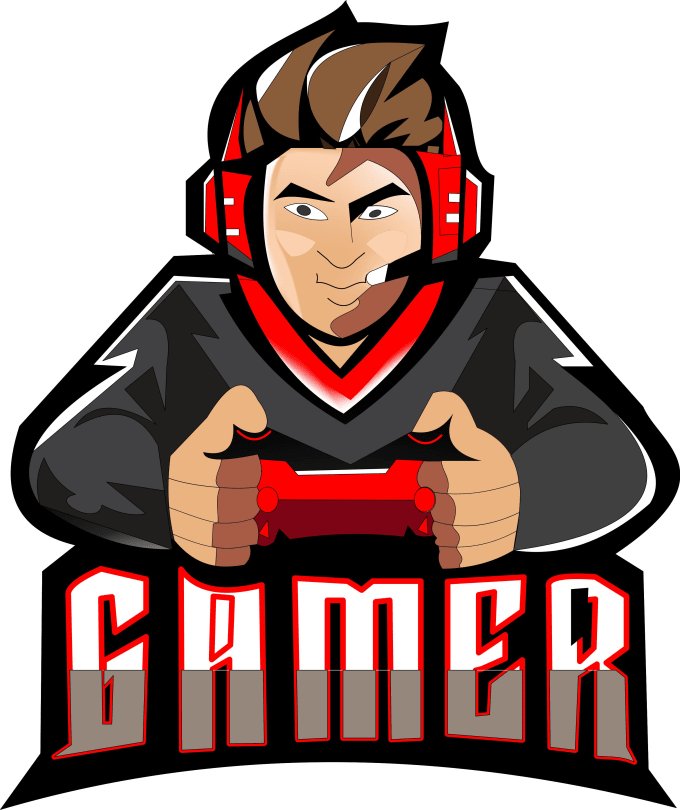The image depicts a highly stylized, cartoony icon of a young man immersed in a video game. With his intense yet happy expression, he looks towards the viewer. His sharp, thick black eyebrows accentuate his long, spiky brown hair, and he's wearing a dark gray, long-sleeved sweatshirt with a red V-neck. Over his ears are bright red gamer headphones, complete with a black microphone positioned near his mouth. His hands grip a red video game controller, with his thumbs poised as if ready to play. The image captures him from the torso up, showing his hunched posture as he leans forward, his arms supported by a desk. Below him, the word "gamer" is prominently displayed in large, white letters outlined in red, conveying the vibrant, angular, and energetic artistic style, similar to a sticker design.